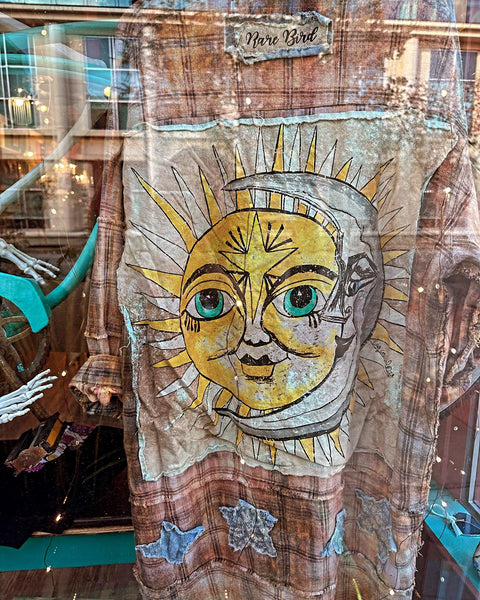This photograph captures a window display featuring a vintage, worn plaid dress in a light brown blush tone with rolled-up sleeves. A badge at the top center of the dress reads "Rare Bird" in red and black print on a curled rectangular tag. The focal point of the dress is a large, square fabric patch sewn onto the back, depicting a vibrant scene with a yellow sun characterized by white and yellow sunrise triangles, black eyebrows, green eyes with black eyelashes, a white nose, yellow lips, and a small star on its forehead. Adjacent to the sun is a crescent moon in gray tones, distinguished by a blue eye, a straight nose, black lips, and a four-sided star in its center. At the bottom of the dress, three blue fabric stars are stitched along the hem. Amid this unique display, there is a distracting reflective glare on the plexiglass window, mirroring a building from across the street, adding to the intriguing complexity of the image. A plastic skeleton foot and hand are visible to the left of the display, adding an eclectic touch to the scene.